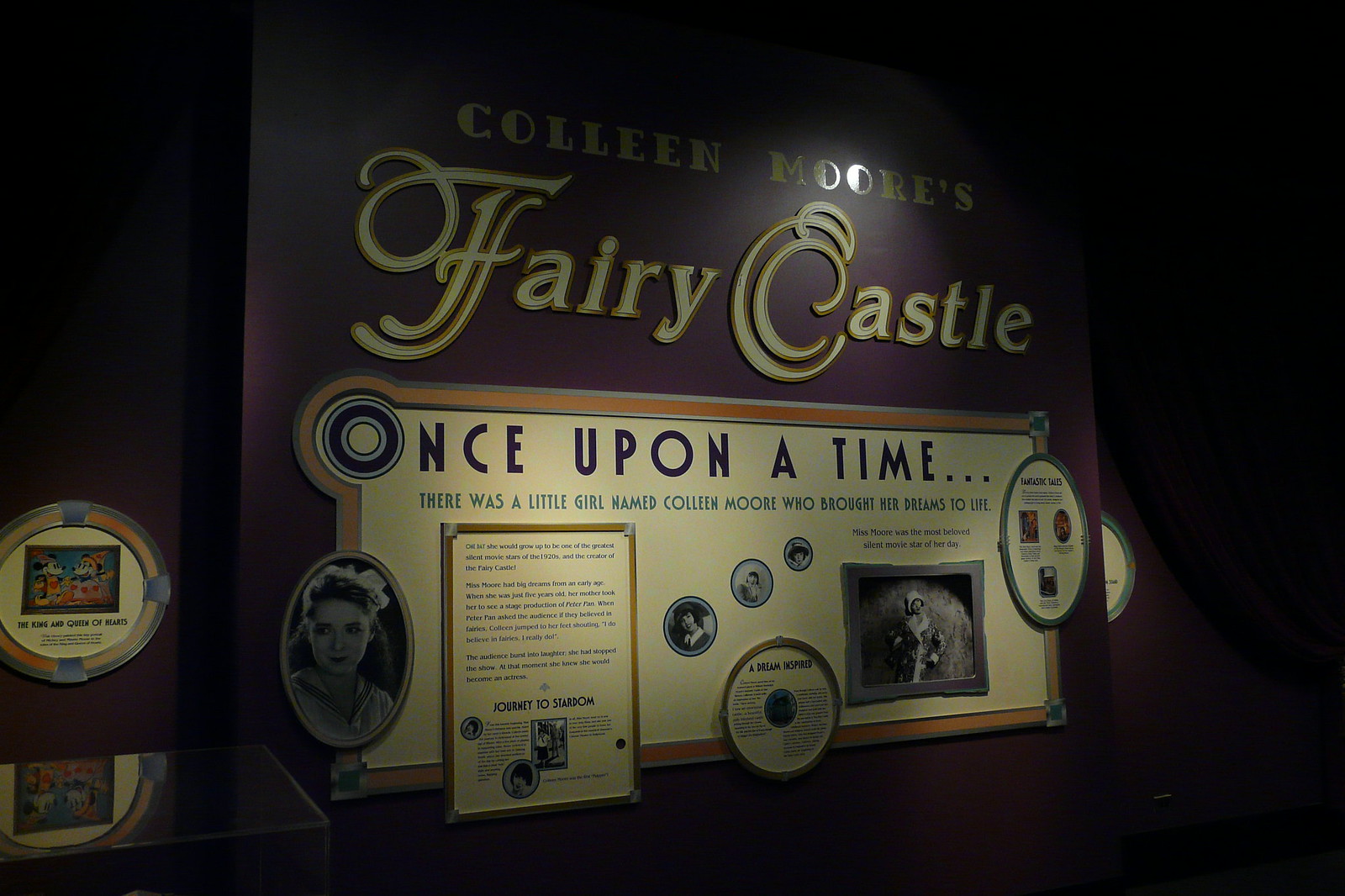The image depicts a dimly lit exhibit sign, likely in a museum, mounted on a deep burgundy or dark purple wall. The exhibit, focused on Colleen Moore's Fairy Castle, is showcased prominently with a stylish dark purple wooden sign. The sign's text is a light yellowish-gold font that declares "Colleen Moore's Fairy Castle" at the top. Below, it transitions into a large light yellow rectangle with an orange frame. Here, in bright purple font, it opens with "Once upon a time..." followed by blue font that reads, "there was a little girl named Colleen Moore who brought her dreams to life." The exhibit also features various black and white photographs and framed objects surrounding the main text, with images that appear to be from the 1930s or 1940s, including several in ovals and circles. The room is dark, enhancing the visual focus on the illuminated sign and the nostalgic photographs, which portray elements of Colleen Moore’s life and her whimsical achievements.